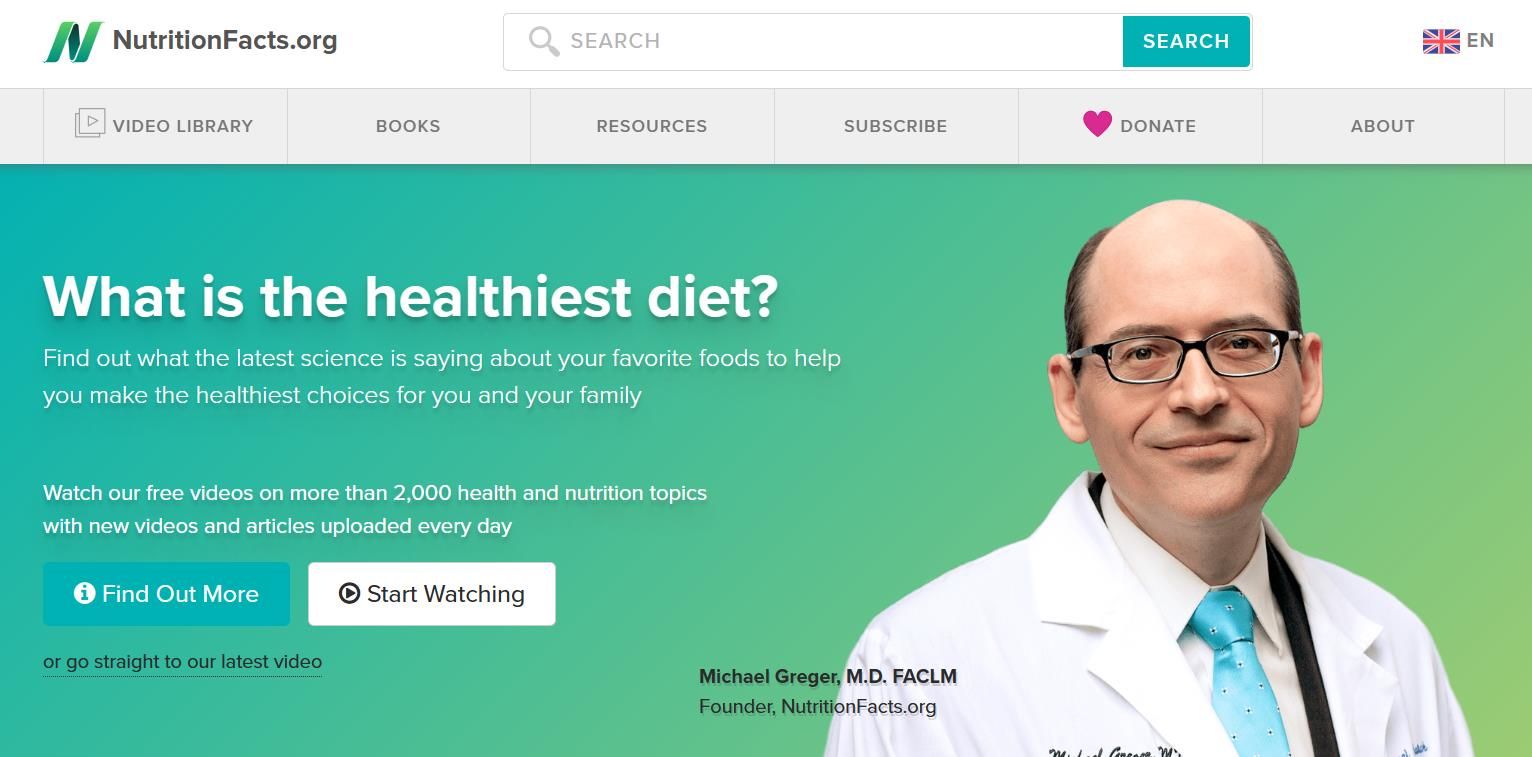The homepage of NutritionFacts.org displays an organized and informative layout that welcomes visitors with various features and resources. At the top, a navigation bar offers links to a video library, books, resources, options to subscribe, donate, and information about the organization. The centerpiece of the page is a prominent, colorful banner. This banner features a rectangular, gradient background transitioning between green and blue hues. Within this rectangle, white text poses the question: "What is the healthiest diet?" and invites users to "Find out what the latest science is saying about your favorite foods, make the healthiest choices for you and your family." 

The banner further encourages visitors to "watch our free videos on more than 2,000 health and nutrition topics," highlighting that new videos and articles are uploaded every day. A call-to-action button, placed within a white square, reads "Start Watching" or offers the option to go directly to the latest video.

In the lower section of the banner, Dr. Michael Greger, MD, FACLM, the founder of NutritionFacts.org, is prominently featured. Dr. Greger, dressed in a white lab coat and a light blue tie with a subtle pattern, is seen looking forward with a slight smirk on his face. He wears glasses and his short dark hair is neatly styled. His collar is white, and a stethoscope is draped around his neck, emphasizing his medical expertise.